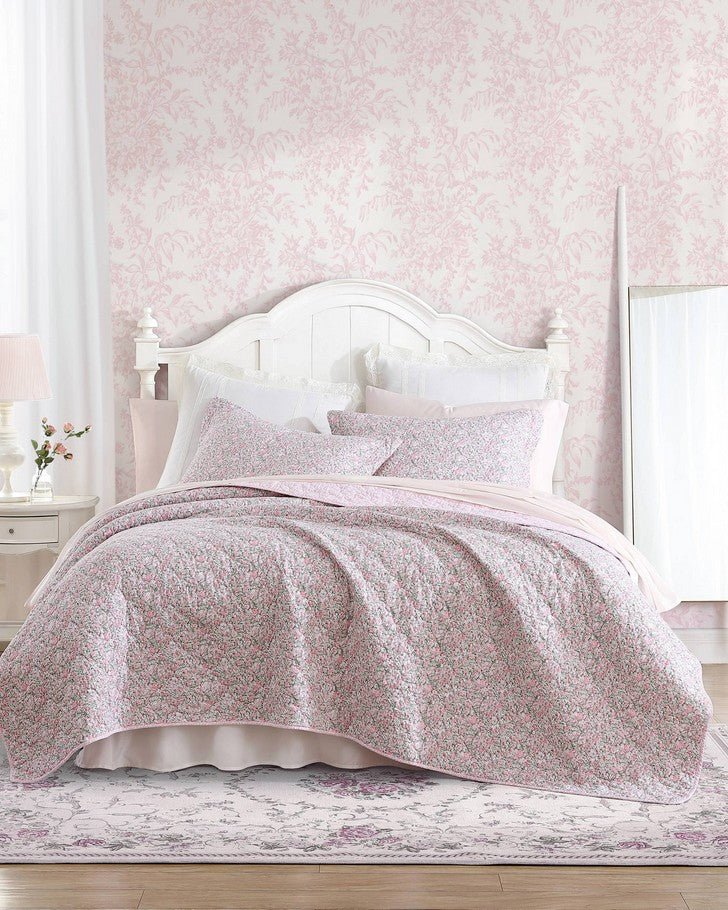The photograph is an indoor, naturally lit, rectangular image likely suited for a catalog or magazine. It portrays a bright, predominantly white bedroom scene. The floor is made of light brown horizontal wood slats, partially covered by a white rectangular rug adorned with pink flowers and green vines. The central focus of the image is a tall bed with a white, beveled wooden headboard. The bed is dressed in a quilt or bedspread that features a delicate pattern of pink and green flowers. Complementing the bedspread are six pillows: two white shams, two light pink shams, and two pillows matching the floral bedspread.

The walls are adorned with white wallpaper featuring a subtle pattern of pink flowers, contributing to the room's cohesive floral theme. To the left of the bed, there is a white end table holding a white lamp and a small clear glass with a pink flower. White curtains frame the left side of the room, while on the right, there is a partially visible cabinet or another white curtained area. A white bed skirt peeks out from beneath the tightly made bed, adding to the overall crisp, clean look of the space.